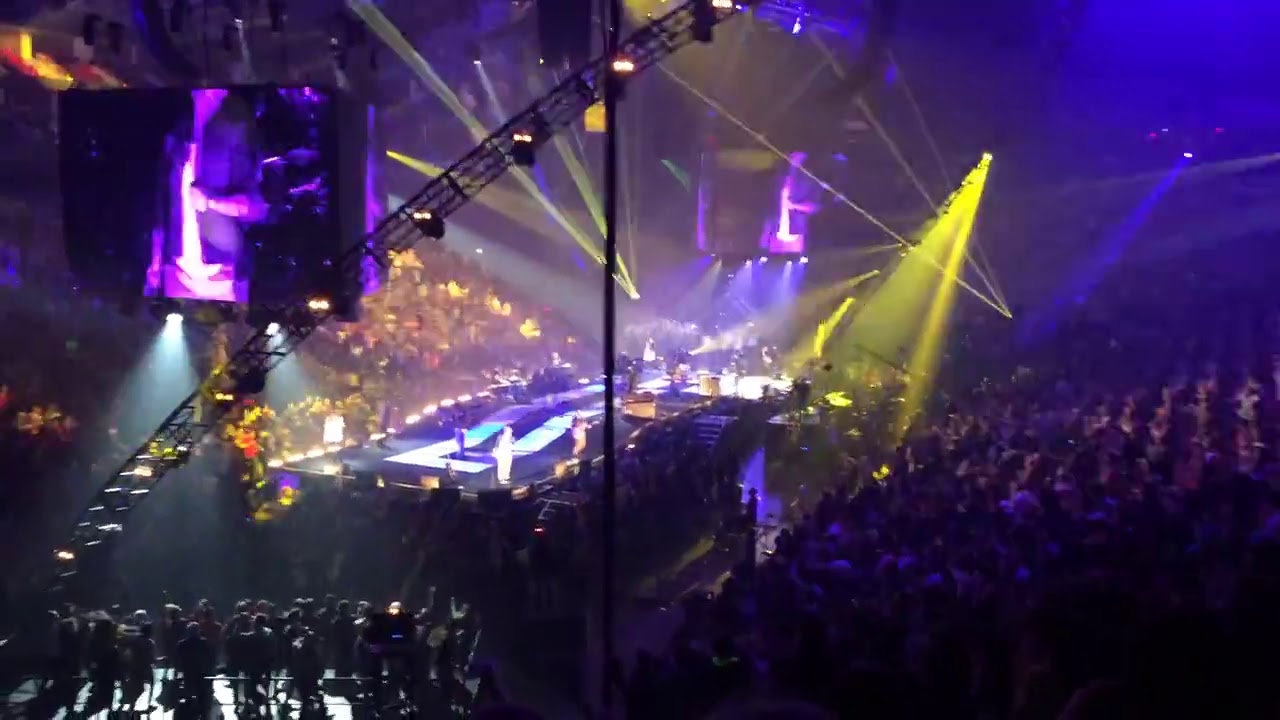The photograph captures a vast indoor venue, likely a concert or a major performance event. In the center, a large stage is flanked by steps and surrounded on all sides by a massive audience, potentially numbering in the thousands. The dark atmosphere is punctuated by vibrant accent lights in shades of purple, blue, yellow, and orange, casting dramatic beams across the scene. Various performers are spread across the expansive stage, with additional people standing off to the side. Suspended from the ceiling is an LED screen visible in the upper left corner, and a crane-like structure with additional lighting rigs extends over the stage, illuminating the area below. Though slightly wooshed out, the image conveys the energy and scale of this packed event.